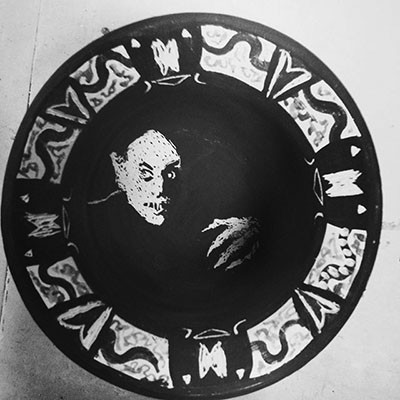A square, black-and-white image with a gray background features a prominent circular design at its center, resembling a collector's plate. This large circular frame, outlined in black, houses an artistic rendition of Nosferatu, the iconic vampire from the 1920s German Expressionist silent film of the same name. Nosferatu's figure, characterized by his pale face covered in artistic spots and his exaggerated, sharp left hand resting on his shoulder, exudes an eerie, monster-like presence. Surrounding Nosferatu within the circular frame are intricate, black-and-white geometric patterns that evoke the essence of Native American or possibly Spanish artistry, adding to the vintage, faded aesthetic of the image.